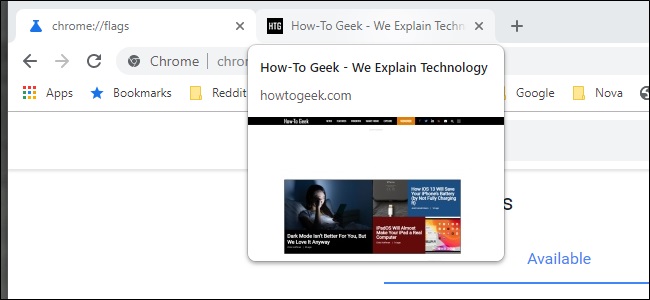This image is a screenshot capturing the interface of Google Chrome with two tabs open. The foremost tab is labeled "chrome://flags", suggesting that the user is viewing Chrome's experimental features settings. However, the URL of this tab is partially obscured by an overlay of the content from the second tab.

The overlay is a preview of a webpage from the second tab. This second tab displays a black square with the bold white letters "HTG", followed by text that reads "How-To Geek: We Explain Technology". Beneath this, in lighter letters, it shows the URL "howtogeek.com". The overlay also provides a miniature view of the webpage layout, which features a black menu bar at the top and various blog posts, each contained within colored square thumbnails.

The overlay of the second tab is designed as a square window superimposed on the first tab, giving a snapshot of what the How-To Geek website looks like while partially blocking the view of the "chrome://flags" tab underneath.